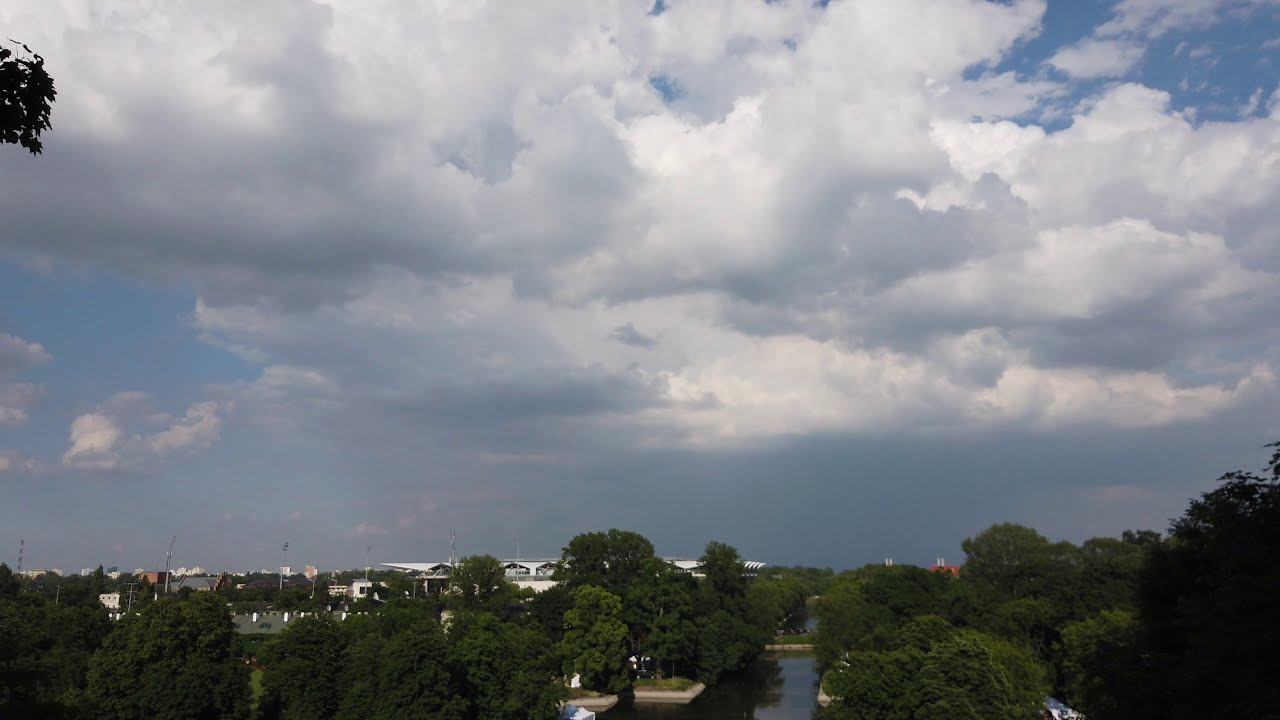This detailed image captures an expansive, cloudy sky, occupying about 70 percent of the frame. The clouds display a mixture of white and gray hues, indicative of rain clouds that haven’t yet released their downpour. They are not overly dark nor fluffy white, rather a mix of impending weather. Beneath this cloud-filled sky, there are green trees dotting the landscape along with a few white buildings scattered throughout the scene. Large telephone poles are visible, interspersed among the greenery and structures. A waterway, possibly a canal, weaves through the town, appearing navigable rather than the result of flooding. The overall photo suggests an outdoor setting, likely captured from an aerial perspective, with the sky above and the assorted trees, buildings, and body of water below, bathed in natural daylight.